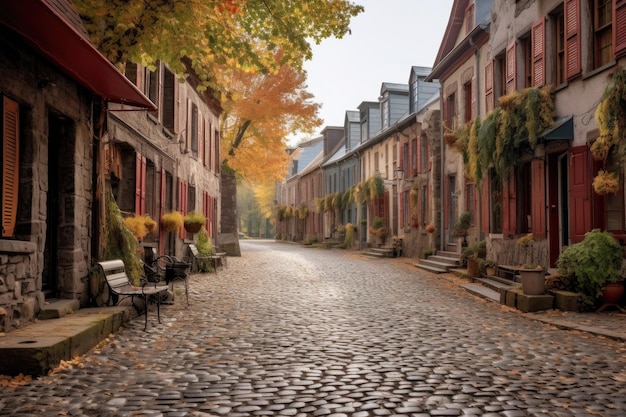This outdoor image, likely captured in the fall, presents a picturesque scene reminiscent of a classic European street or an old-school town. Dominating the center is a wide, cobblestone walkway that narrows as it extends into the background. On both sides of this path, rows of two to three-story houses and buildings line the street. These structures, primarily composed of gray bricks with some white and red accents, feature striking red shutters and doors that harmonize with the overall historic aesthetic. Cement steps lead up to the red entryways on the right-hand side, where potted plants add a touch of greenery. On the left, benches are placed in front of the houses, inviting passersby to sit and enjoy the surroundings. The tops of the buildings display a mix of taller gray rooftops. Overhanging branches with green, yellow, and red leaves hint at the autumn season, while the sky above appears grayish but clear. This array of details paints a vivid picture of a quaint, old-world street scene.